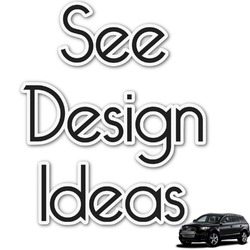This image is an online graphic or sticker featuring the phrase "See Design Ideas" prominently displayed in black font with a white outline, centered on a white background. In the bottom right corner, there is a smaller image of a black car, which resembles a four-door SUV, such as a Range Rover. The car is detailed with distinct features like four doors, a grille, door handles, and glass windows. The font of the text is somewhat playful, reminiscent of Comic Sans.